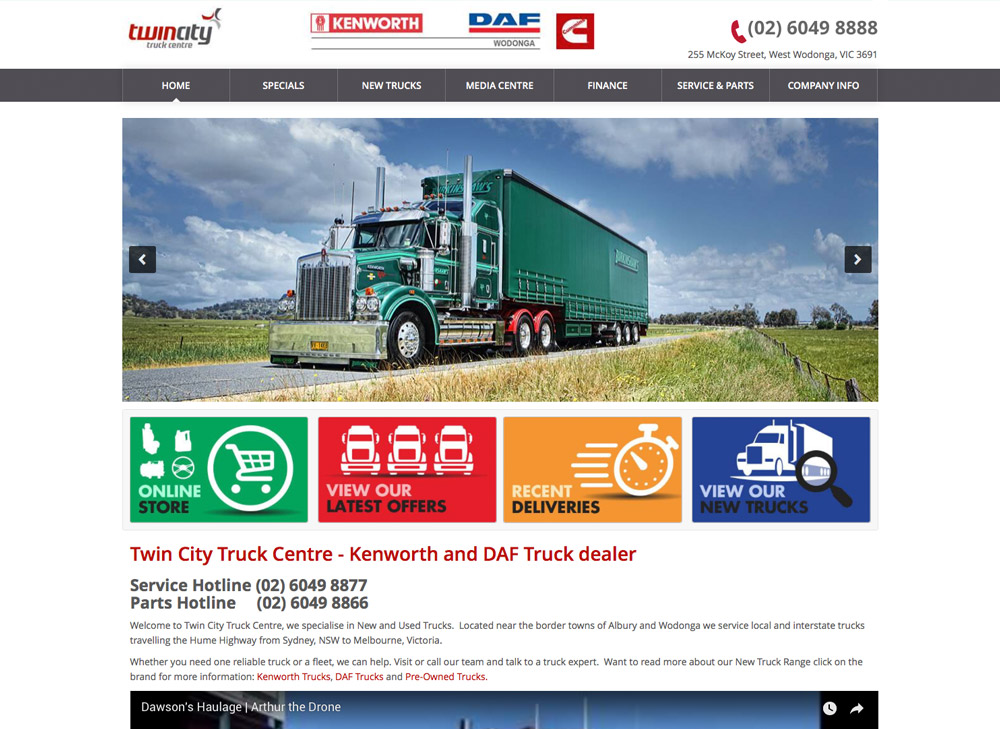This is a screenshot from the website Twinity. The Twinity logo is positioned on the far left side of the header, with "Twin" in red and "ity" in black, creating a single word. Below the Twinity logo, the words "Truck Center" are displayed. Still on the top left side of the header, towards the center, there is a banner featuring the logos of Kenworth and DAF, alongside a "Wodonga" banner and a red box with the letter "C". On the farthest right, there's a telephone number displayed as 026-049-8888 and an address reading "255 McCoy Street, West Wodonga, Victoria 3691."

A black menu bar spans across the header with several tabs: "Home," "Specials," "New Trucks," "Media Center," "Finance," "Service and Parts," and "Company Info." Below the menu bar, the website content features a large slider image depicting a green freight truck driving on a country road.

Directly below the slider image, there are four smaller picture icons. The first icon, in green, says "Online Store" and features a shopping cart image. The second icon, labeled "View Our Latest Offers," shows three white trucks on a red background. The third icon, titled "Recent Deliveries," includes a graphic of a stopwatch. The fourth icon reads "View Our New Trucks" and displays a blue background with a white silhouette of a truck overlaid by a black magnifying glass.

Directly beneath these icons, bold red text reads "Twin City Truck Center, Kenworth, and DAF Truck Dealer," followed by two phone numbers for a service hotline and a parts hotline. Additionally, there are two to three sentences of text where the words "Kenworth trucks," "DAF trucks," and "preowned trucks" are highlighted in red.

At the bottom of the page, the footer contains "Dawson's Haulage" and an author citation on the left side, and on the right side, there are icons of a clock and an arrow.